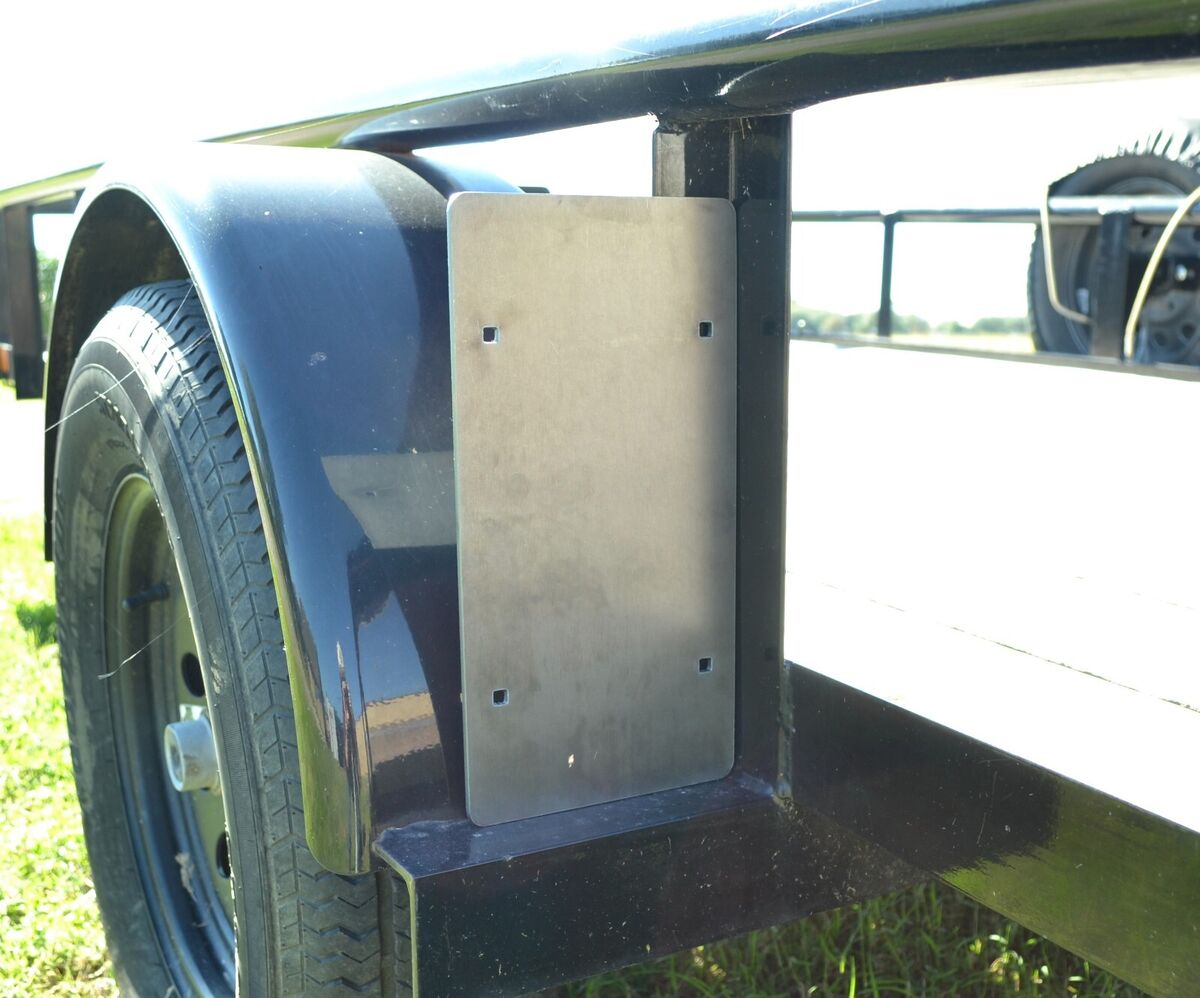This image is a detailed close-up of a heavy-duty flatbed trailer set in a bright, open field under a pale sky. Dominating the left-hand side of the photograph is a very large rubber tire with a silver rim. The hubcap or the area bordering the tire is a dark blue or black metal, with a small patch of green near the fender. A vertical rectangular metal plate is positioned in front of the wheel, and there's a bar extending from above the wheel, shaded in light green and black. The trailer bed stretches to the right side of the image, empty and ready for loading. The bright green grass beneath the vehicle glistens under the sunlight, illuminating the scene. Surrounding the trailer are fields that extend into the distance, with a faint sight of a mountainous structure on the horizon. The vehicle's metal parts are particularly shiny, reflecting the sunlight and nearby objects, while delicate spider webs hang off the wheel, adding a touch of intricate detail.